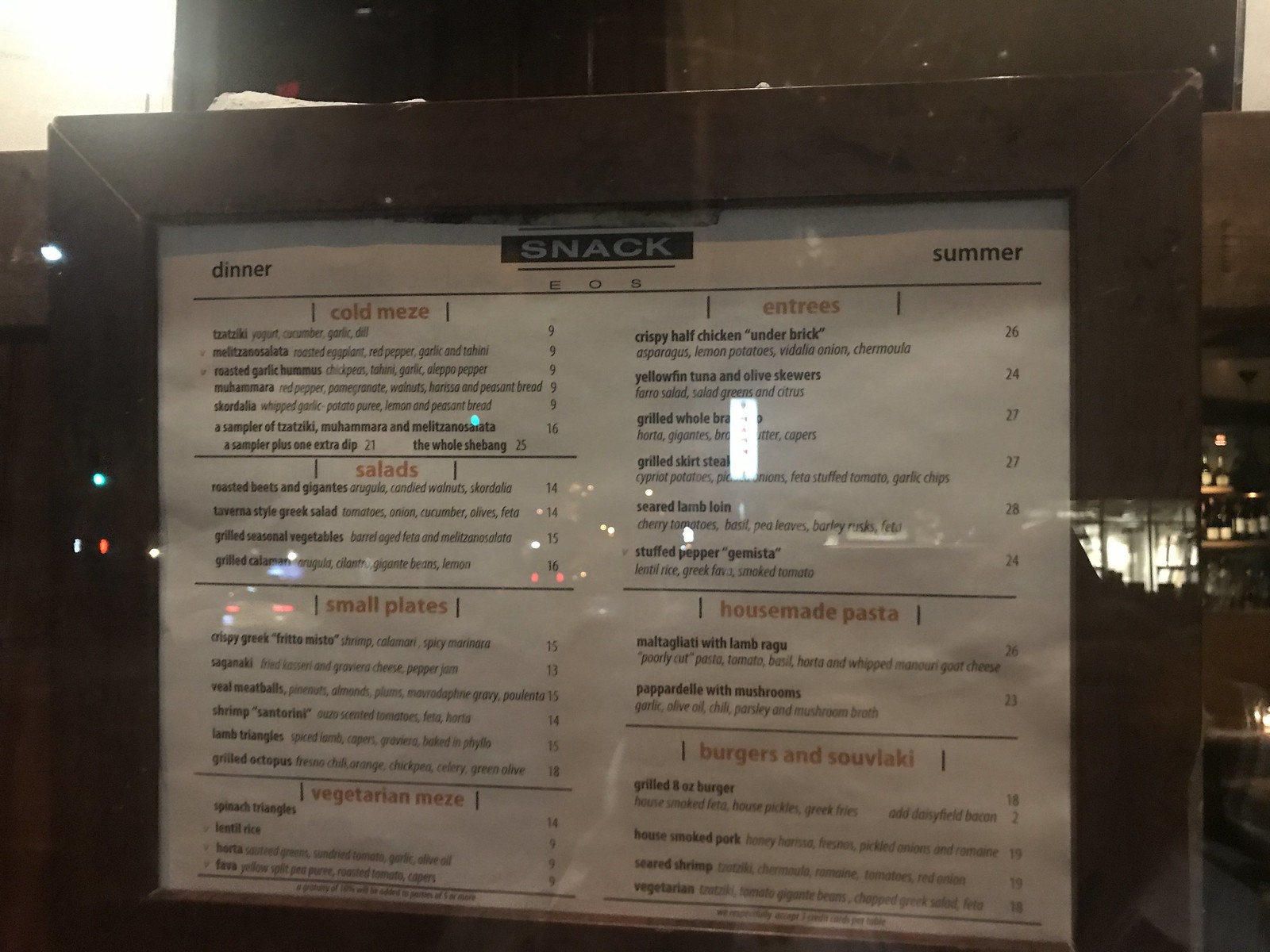This photograph captures a restaurant menu through a window, resulting in the image being somewhat obstructed and challenging to read due to reflections. The reflections reveal an outside cityscape with advertising signs and passing cars, indicating the camera is capturing the urban activities behind the photographer. The menu, enclosed in a black frame that shows signs of wear and set behind a glass cover, dominates approximately 90% of the frame. In the distant background, inside the establishment, a bar area with bottles is partially visible against a white wall.

The menu itself features a clean design with a predominantly white background, accented by black borders and text, accompanied by some red text. At the top, the headings "Dinner" on the left and "Summer" on the right frame the central word "Snack," which is highlighted in a black-bordered white lettering, with the letters "E O S" delicately placed underneath.

The left column of the menu is divided as follows:
- "Cold Meze" (Meze spelled M-E-Z-E) with a list of several items.
- "Salads" with four different options.
- "Small Plates" in red, enumerating around six dishes.
- "Vegetarian Meze" listing four selections.

The right column presents the following sections:
- "Entrees" in red, detailing six different main courses.
- "House-made Pasta" with two varieties.
- "Burgers and Souvlaki" listing four choices.

This detailed description provides a snapshot of both the menu and its context within the bustling city environment, offering insight into the restaurant's eclectic offerings and ambiance.